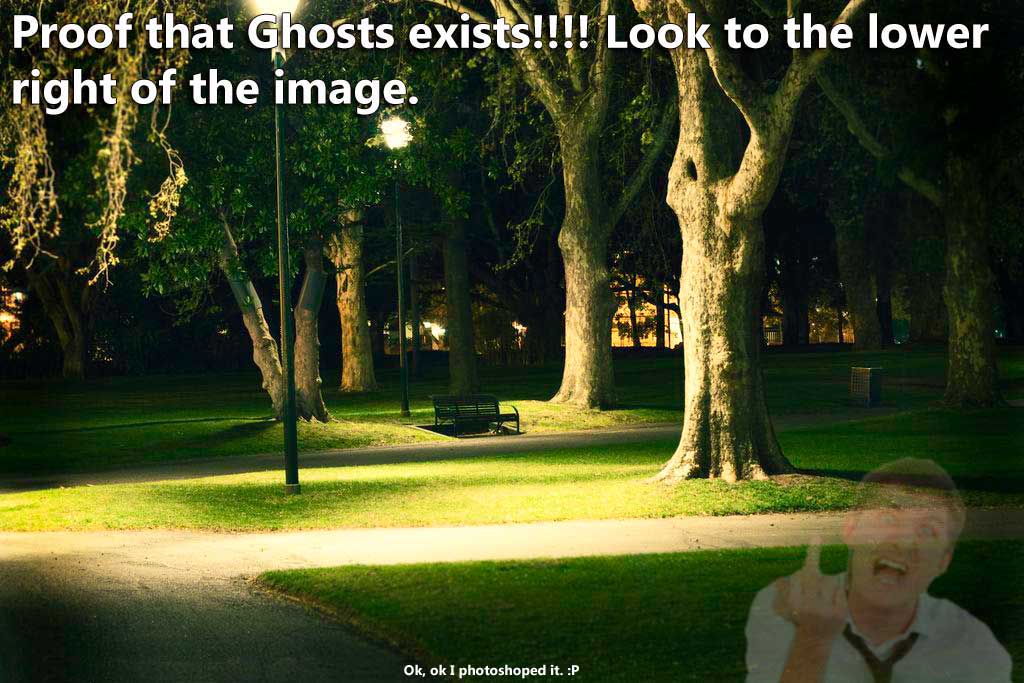The image depicts a serene, empty park at night, resembling the grounds of a university campus. The park features concrete walkways and paved footpaths interspersed with old, tall trees with drooping branches. Lampposts with black poles and lit lamps are positioned at intervals along the pathways, illuminating the scene. Park benches and trash cans line the walkways, and green grass extends across the area.

In the upper part of the image, white text reads, "Proof that ghosts exist." In the lower right corner, there is a semi-transparent overlay of a young man with a crazed look on his face, wearing a white collared shirt and black tie, flipping the middle finger at the viewer. This figure appears ghostly and faded, enhancing the eerie atmosphere. In small text at the bottom center of the image, it humorously reads, "Okay, okay, I photoshopped it," accompanied by a tongue-out face emoticon, suggesting that the ghostly figure was digitally added to the scene.